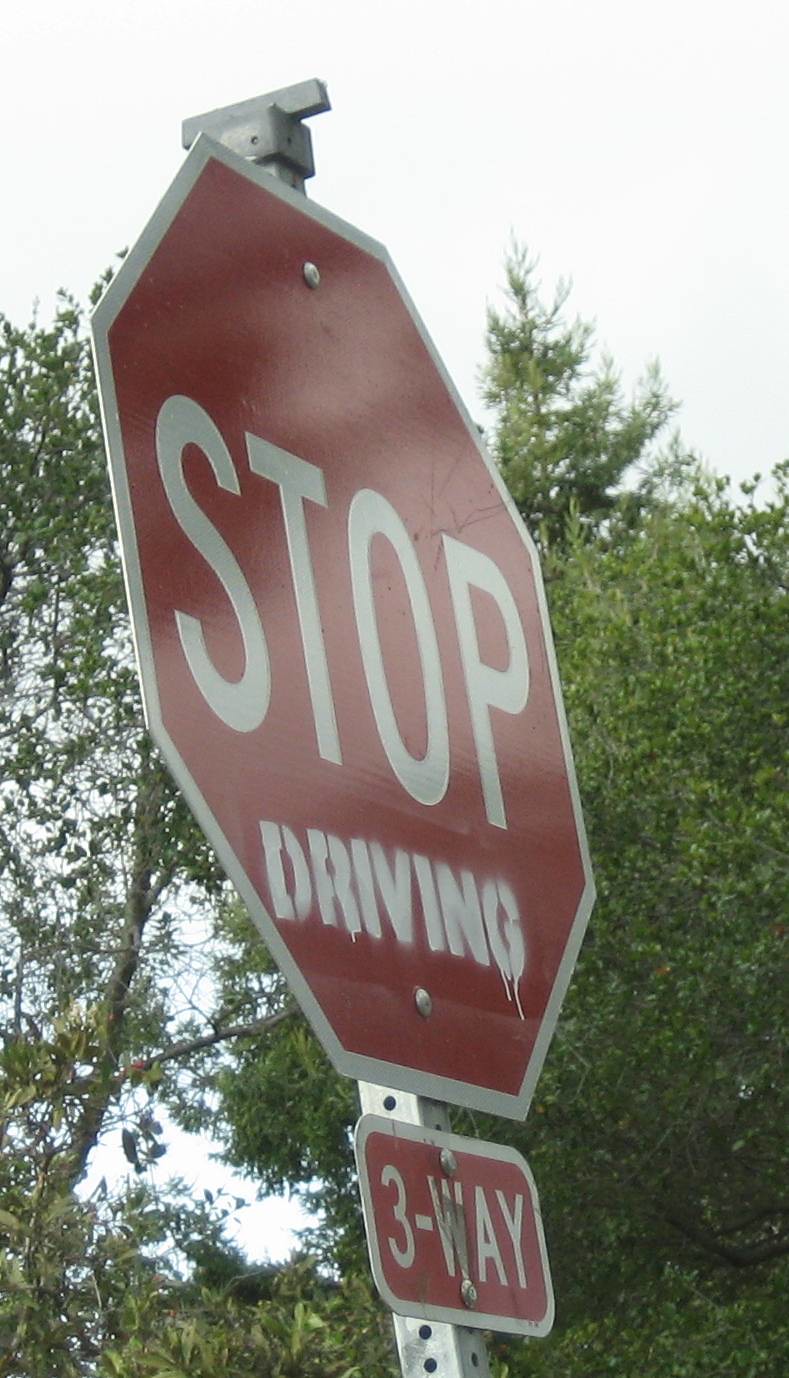This is a detailed photograph of a three-way stop sign, prominently positioned at the center of the frame. The stop sign bears the stencil-spray-painted text "STOP DRIVING," with the word "driving" noticeably added beneath the word "STOP." Directly below the main sign, a smaller plaque indicates "three-way," confirming the type of stop. The sign is mounted on a metal pole, and the scene is set amidst tall trees on either side, suggesting a roadway environment. The photo features a diverse color palette including green, blue, red, white, and silver. The angle of the shot appears to be taken from below and to the left of the sign, adding an artistic tilt that enhances the visual interest. The surroundings imply that the photographer likely exited their vehicle to capture this unique and compelling image.